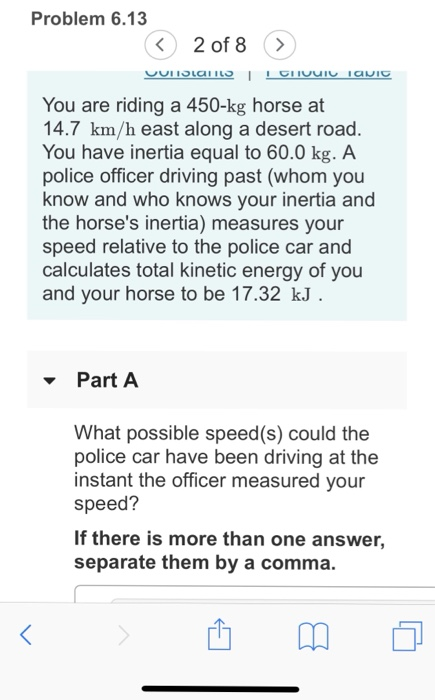This mobile screenshot appears to be from a homework or educational app displaying Problem 6.13. At the top of the screen, there is an indicator showing "Page 2 of 8" with encircled arrowheads on either side for navigation. 

The main content area features a pale blue text box which reads: "You're riding a 400-kilogram horse at 14.7 kilometers per hour east along a desert road. You have inertia equal to 60 kilograms. A police officer driving past—whom you know and who knows your inertia and the horse's inertia—measures your speed relative to the police car and calculates the total kinetic energy of you and your horse to be 17.32 kJ."

Below the problem statement, within a pale gray rectangle, is a section labeled "Part A" which includes a dropdown menu. The accompanying question posed in black font on a white background is: "What possible speeds could the police car have been driving at the instance the officer measured your speed? If there is more than one answer, separate them by a comma."

At the bottom of the screen, the user interface includes:
- A blue left arrow,
- A grayed-out right arrow,
- A share icon depicted as a square with an arrow pointing upwards,
- An open book icon that likely represents a reading list function, 
- Two overlapping squares, possibly indicating the copy function.